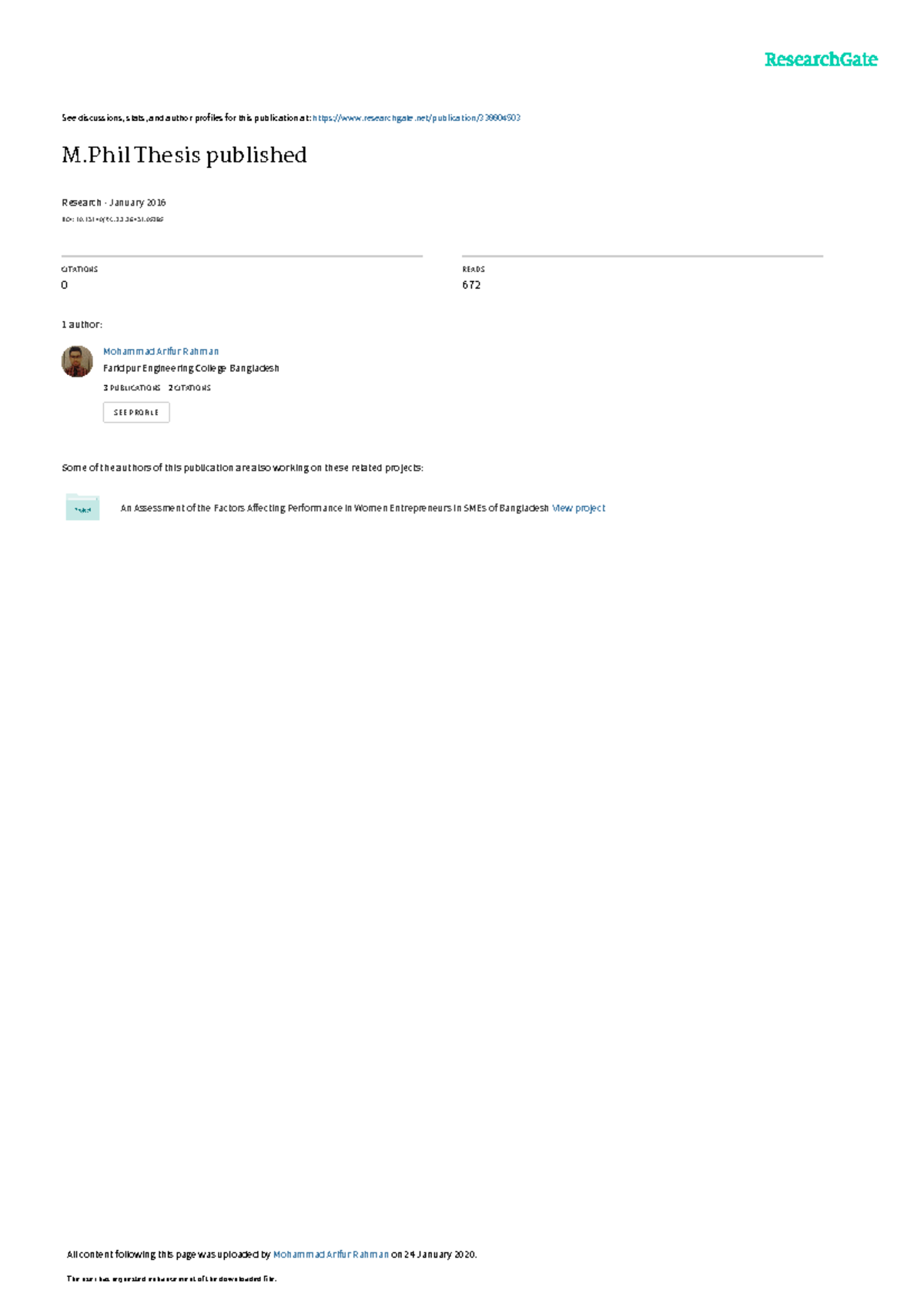This image is an excerpt from a thesis published on ResearchGate, a scholarly platform. The top-right corner shows the ResearchGate logo, with "Research" and "GATE" in teal, and both 'R' and 'G' capitalized. Below, the text reads: "See discussions, stats, and author profiles for this publication at" followed by a website link. The document is an M.Phil Thesis published in January 2016, indicated near the top-middle. Faint numbers and letters are scattered throughout, likely metadata or identifiers. A faint gray line runs horizontally across the document but is interrupted halfway and resumes mid-page to the right. Below this line, the statistics show "Citations: 0" and "Reads: 672." A profile picture of the sole author, Mohamed Afar Rahman, appears beside the text. The bottom section of the page remains largely blank, stating that all following content was uploaded by Mohamed Afar Rahman on January 24, 2020.